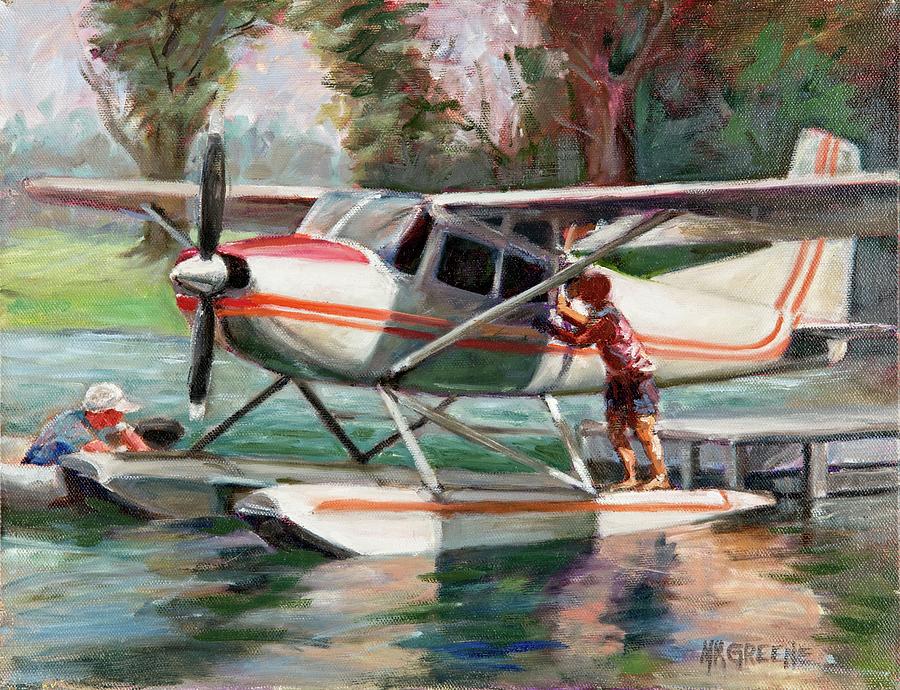This detailed oil painting by M.R. GREEN, signed in the lower right corner, captures a serene lakeside scene featuring a single-engine, Cessna-type pontoon airplane docked on the water. The white aircraft is adorned with distinctive orange stripes along the sides and up to the middle of the tail fin. The pontoons, similarly adorned with an orange stripe across the top, rest gently on the colorful water, which reflects hues of blue, green, and tan.

In the foreground, a boy in shorts and a tropical shirt stands on the left pontoon, near the back window of the cockpit, appearing to either enter or exit the plane as he grasps the door. On the right pontoon, towards the front of the plane, a man in a blue shirt and white baseball cap sits in a dinghy with an engine, either rowing or maneuvering the boat to or from the aircraft. The man looks relaxed, leaning out of the dinghy, his actions partially obscured by the pontoons.

The background of the painting reveals lush green hills and a forested area, enhanced with impressionistic strokes that create a sense of depth. Trees in various shades of green transition into muted tones, providing a soft, distant view. Above, a sky filled with pinks and blues adds a tranquil ambiance to this picturesque lakeside setting.